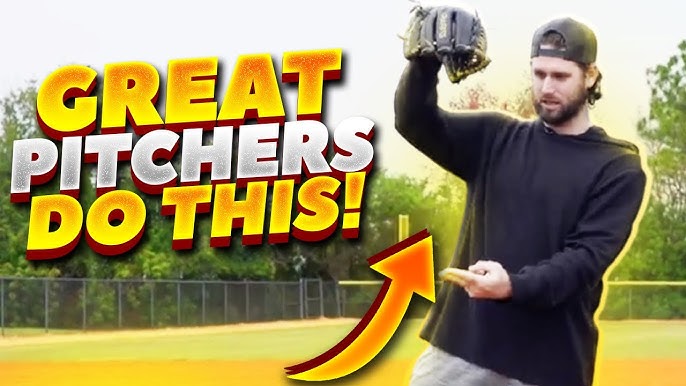This image, which appears to be designed as a thumbnail for a YouTube video, features bold, exuberant text that reads, "Great pitchers do this!" The words "Great" and "do this" are highlighted in a bright gold-orange color, while "pitchers" stands out in a striking silver hue. Dominating the right side of the image is a young man, who is white, with facial hair, and is wearing a black, backward baseball cap. He sports a black long-sleeve hoodie and gray pants. His stance turns slightly left, with his right hand, donned with a baseball glove, raised at head height, palm down, and his left hand pointing at the arrow. This large, illustrated orange arrow starts from the bottom middle of the picture and directs the viewer's eye towards the man. The backdrop showcases a chain-link fence with yellow padding along the top, forming a corner in the center, and a partially visible gate. In the background, there are faintly visible trees against a whitish sky, framing the scene on a sports field.